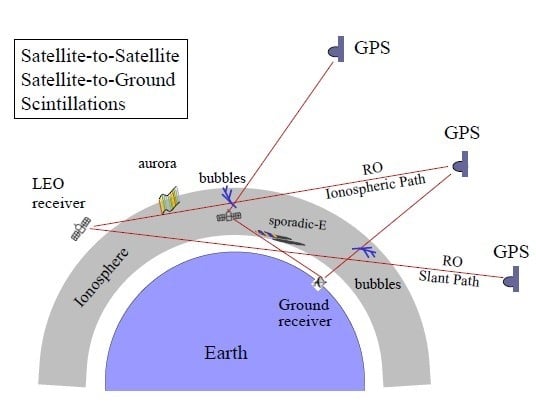The image, titled "Satellite to Satellite, Satellite to Ground, Scintillations," is a detailed diagram illustrating a network of satellites and their interactions with the Earth and the ionosphere. At the center is a purple semicircle labeled "Earth," surrounded by a white outer edge and a thicker gray edge. The gray perimeter is marked on the left as "ionosphere" and on the right as "bubbles."

A rectangular information box at the top left contains text describing "satellite-to-satellite," "satellite-to-ground," and "scintillations." The diagram shows intricate lines and arrows depicting the paths of GPS signals from three GPS satellites situated on the right side. These signals interact with various receivers, including a Low Earth Orbit (LEO) receiver on the left and ground receivers.

Additional labels in the diagram include terms such as "aurora," "bubbles," "ground receiver," "RO," "slant path," "ionospheric path," and more, which describe different pathways and interactions of satellite signals within and through the ionosphere to various earth-based receivers. The overall graphic encapsulates multiple layers of atmospheric interaction, with the ionosphere and its sporadic activity playing a central role in the transmission paths of satellite communications.